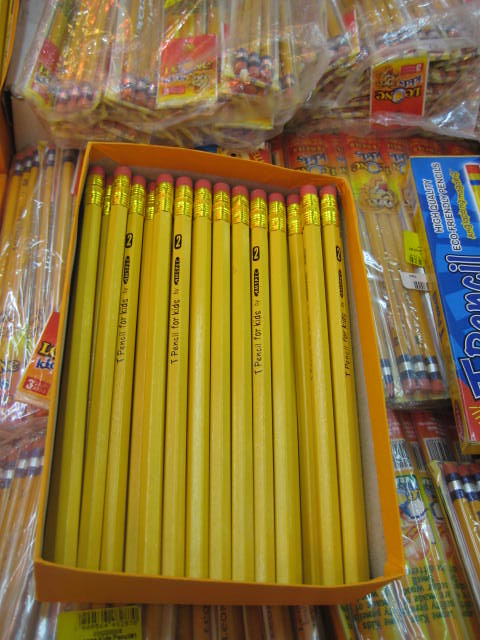The image is a color photograph taken from above under artificial lighting, giving it a yellowish hue. At the center is a large orange rectangular cardboard box without a lid, neatly filled with around 20 to 30 unsharpened yellow pencils. Each pencil has a gold-colored ferrule with a red eraser. The pencils have black text printed on them addressing them as "pencil for kids." The box is resting on a substantial pile of more yellow pencils, which are wrapped in clear plastic packaging, seemingly in packs of three. Reflections from the light source above create a slight glare on the plastic. There's an indecipherable label on the right side of the box, and the image includes some lion-like logo or design on the packaging, further adding to the scene's detail. The setting appears to be either a store or a pencil factory.